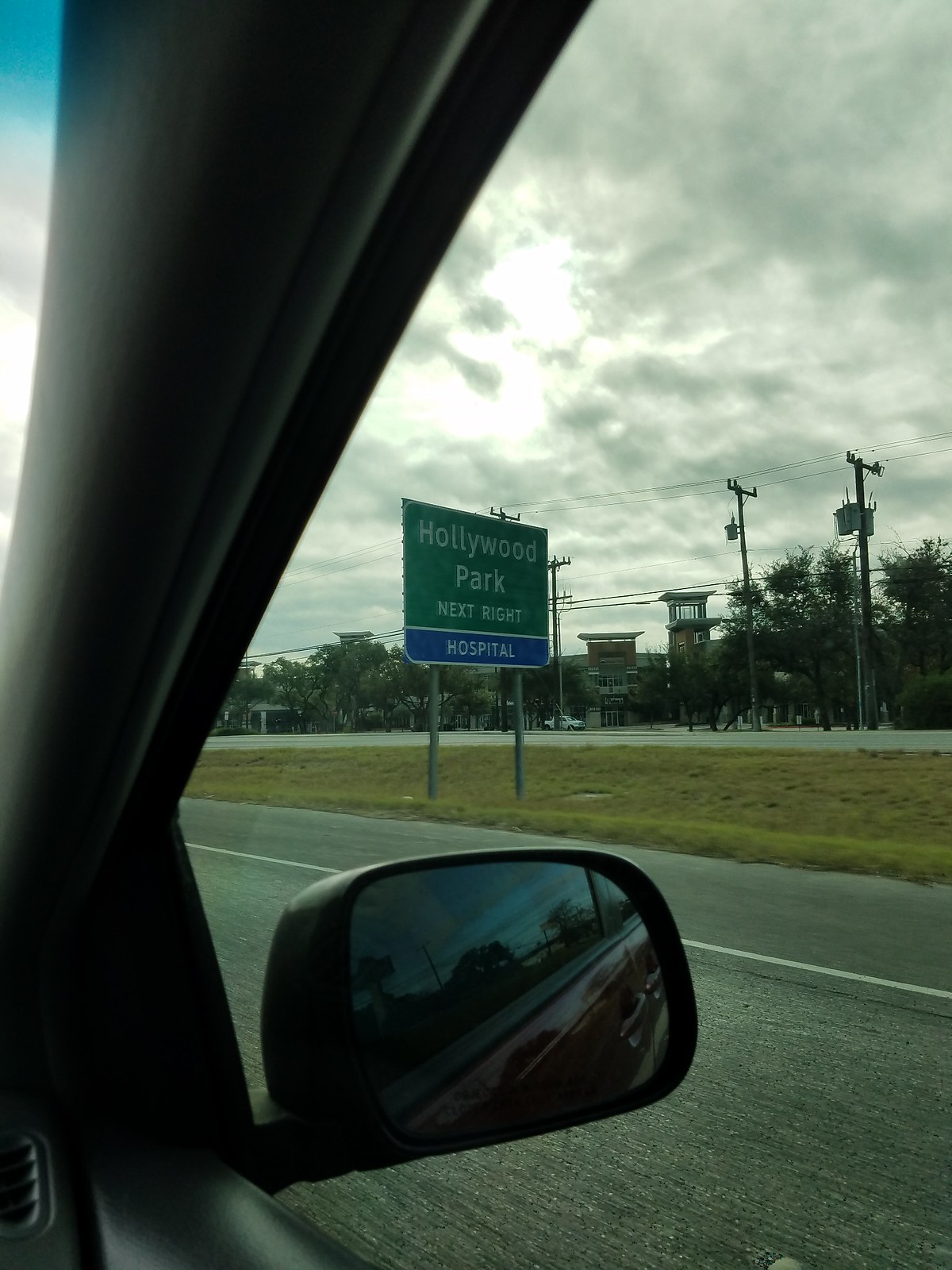A first-person point of view image is taken from the right-hand passenger seat of a car. The interior of the car is partially visible, lined with black rubber material. A small portion of the dashboard, crafted from wood, is seen at the top and middle left of the photograph. The main focus is the view through the side window, directly facing a road sign situated in a grassy median dividing two lanes of traffic. 

The sign consists of two sections: the larger top section is green with white text reading "Hollywood Park, next right." Beneath it, there is a smaller purple rectangle sign that simply states "hospital" in white text. The sky above is covered with grey clouds, creating an overcast atmosphere. In the background, we can see power lines, power poles, and a building with a truck parked in front of it, adding depth to the suburban landscape.